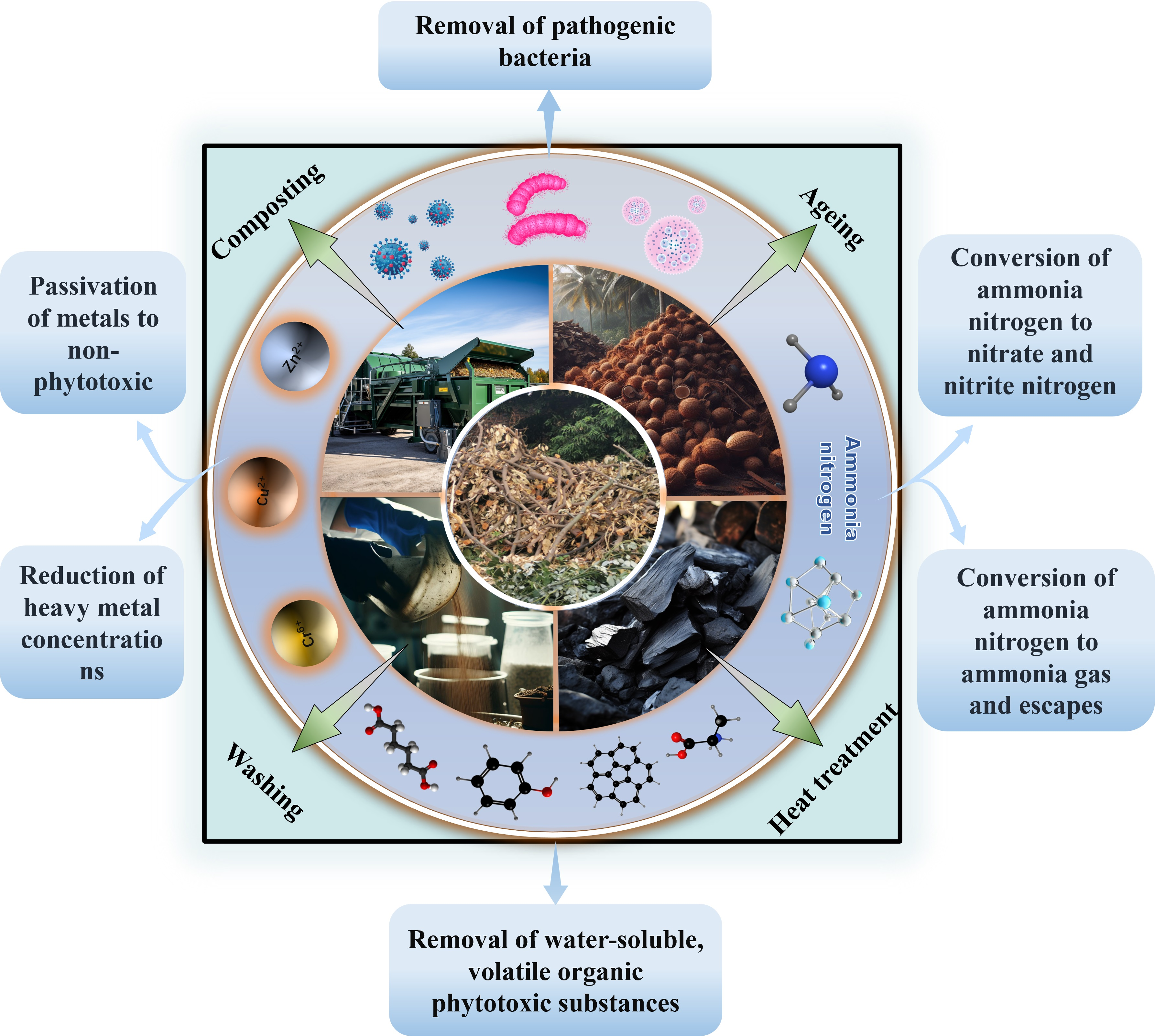The image is a full-color promotional educational diagram set against a white background. At its core, a smaller white circle is encased within a larger blue square, which is surrounded by a series of additional blue squares and rectangles. This central circular chart is divided into four sections, labeled "composting," "aging," "washing," and "heat treatment," each depicting various farming and industrial processes, including the use of a tractor and close-ups of hands wearing gloves washing materials. Surrounding the central diagram, numerous captions detail the scientific aspects, such as the "removal of pathogenic bacteria," "conversion of ammonia nitrogen to nitrate and nitrate nitrogen," "reduction of heavy metal concentrations," and the "passivation of metals to non-phytotoxic forms." The diagram also highlights images of bacteria, cells, and molecules, with annotations explaining steps like the transformation of substances during these processes. Despite its complexity, the brightly lit, detailed images make the intricate information more accessible.